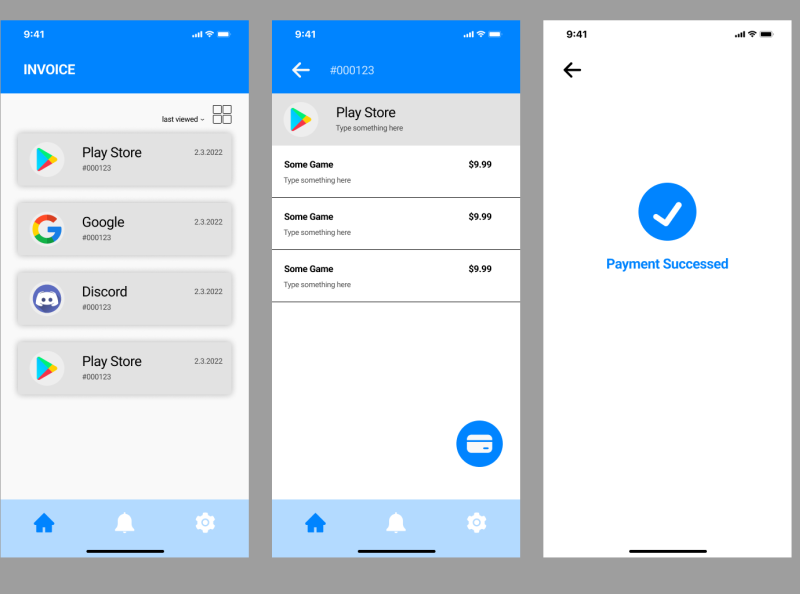The image comprises three separate phone screenshots, all captured at 9:41 AM and depicting various screens related to an invoice and payment process. 

1. **First Screenshot: Invoice Page**
   - **Time & Connectivity**: The status bar indicates full network bars, active Wi-Fi, and full battery.
   - **Layout**: The screen shows an invoice page with white text on a blue header at the top.
   - **Navigation Bar**: At the bottom of the screen are the Home, Notification, and Options buttons.
   - **Recent Views**: Displays the last accessed apps which include Play Store, Google, Discord, and the Play Store again.

2. **Second Screenshot: Payment Details**
   - **Time & Connectivity**: Similar status bar details with full bars, Wi-Fi, and battery.
   - **Screen Elements**: Features a back arrow with the number 00123.
   - **Content**: A list of items labeled "some game" each priced at $9.99.
   - **Icons**: Contains a small white credit card icon and a blue bubble at the bottom right corner.
   - **Navigation Bar**: Home, Notifications, and Settings buttons are present.

3. **Third Screenshot: Payment Confirmation**
   - **Time & Connectivity**: Consistent status bar features, full bars, Wi-Fi, and battery.
   - **Screen Elements**: A black back button and a blue bubble with a white check mark indicating a payment confirmation.
   - **Text**: Initially reads "Payment Successed," but is corrected mid-description to "Payment Succeeded."
   - **Navigation Bar**: Includes Home, Notifications, and Settings buttons.

Overall, these screenshots display a user navigating through their payment history and invoice details on their phone, with an annotation pointing out a typographical error in the payment confirmation message.